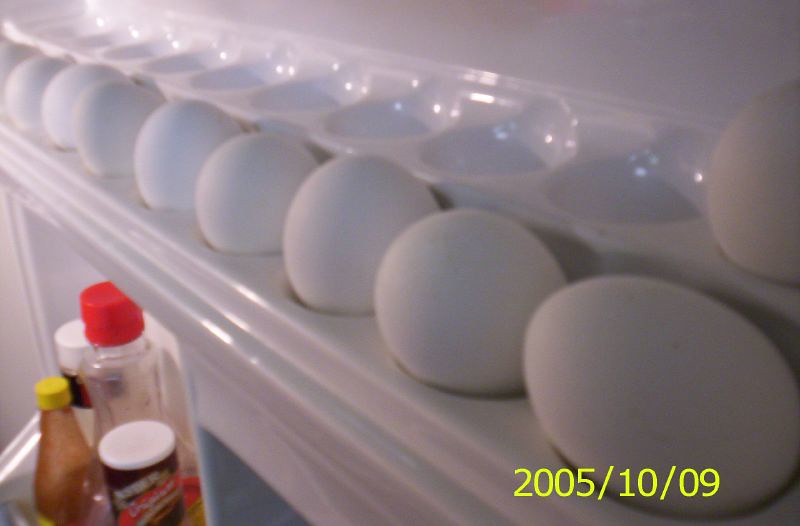This photograph, dated October 9, 2005, captures the interior of a white refrigerator door. Prominently featured is a plastic egg tray with multiple depressions designed for holding eggs. The tray displays nine white eggs: eight arranged neatly in the bottom row and one sitting alone in the top row, highlighting the different levels of the tray. The background emphasizes the monotone white of the refrigerator, creating a sharp contrast with the eggs. Below the egg compartment, a lower shelf showcases several condiments, including identifiable bottles of ketchup or hot sauce, pancake syrup, and salad dressings. The yellow date stamp in the lower right corner confirms the photograph's time frame. The strategic perspective of the image directs attention primarily to the eggs while offering a glimpse into the neatly organized condiments below.